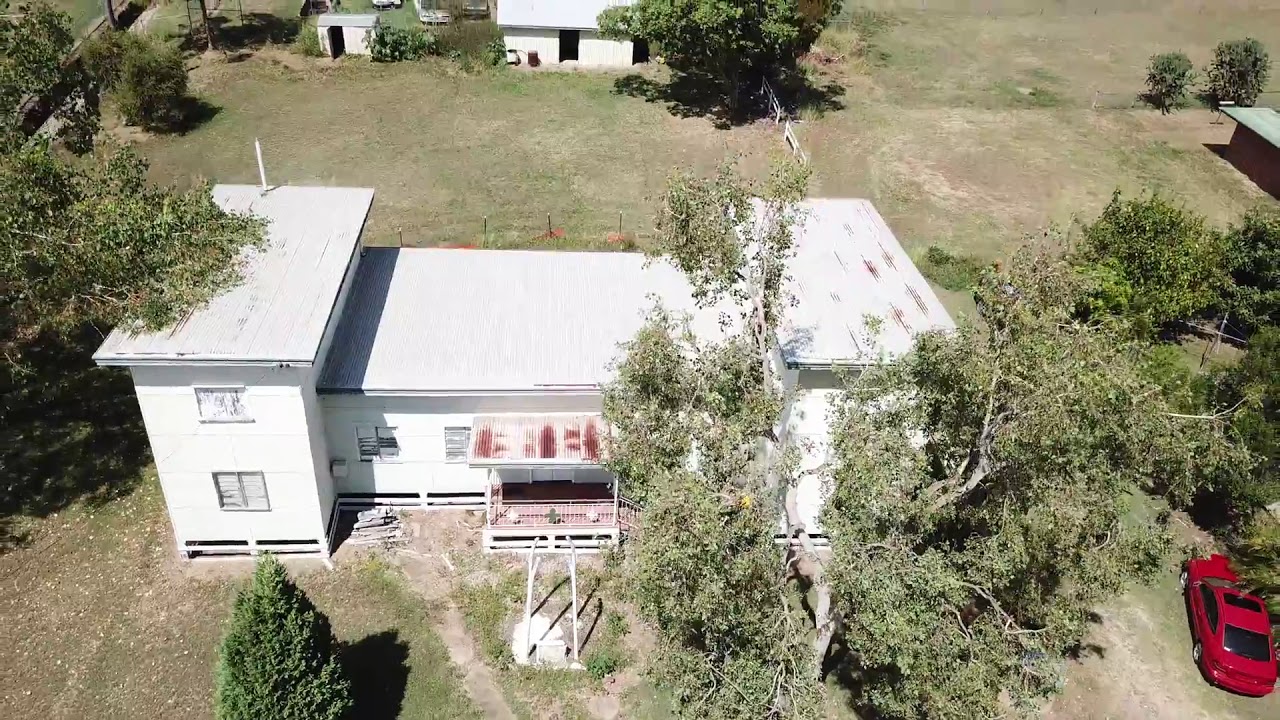This aerial view captures a spacious and intricately structured white home. The house is distinctly divided into three sections: the central section is single-story, flanked by two-story sections on either side. The rooftop is a mix of white and rusted patterns, with numerous windows adorning each part of the home. A wooden deck extends from the house, providing a cozy outdoor space. Surrounding the home, lush green fields stretch out, interspersed with patches of sun-worn grass where dirt shows through. To the back of the field, a couple of white sheds, possibly an old garage or additional storage, are seen. Tall, green trees, some with sun-bleached foliage, create a natural border around the property, with some partially concealing the rear sections of the house. The foreground of the image features a red sedan with a sunroof, parked in the lower right corner, presumably in the driveway. Scattered shadows from the trees provide a sense of depth and highlight the sunlight bathing the rural scene. The wider area includes other structures and hints of a nearby street or waterway to the left, emphasizing the property's location in a serene, rural neighborhood.